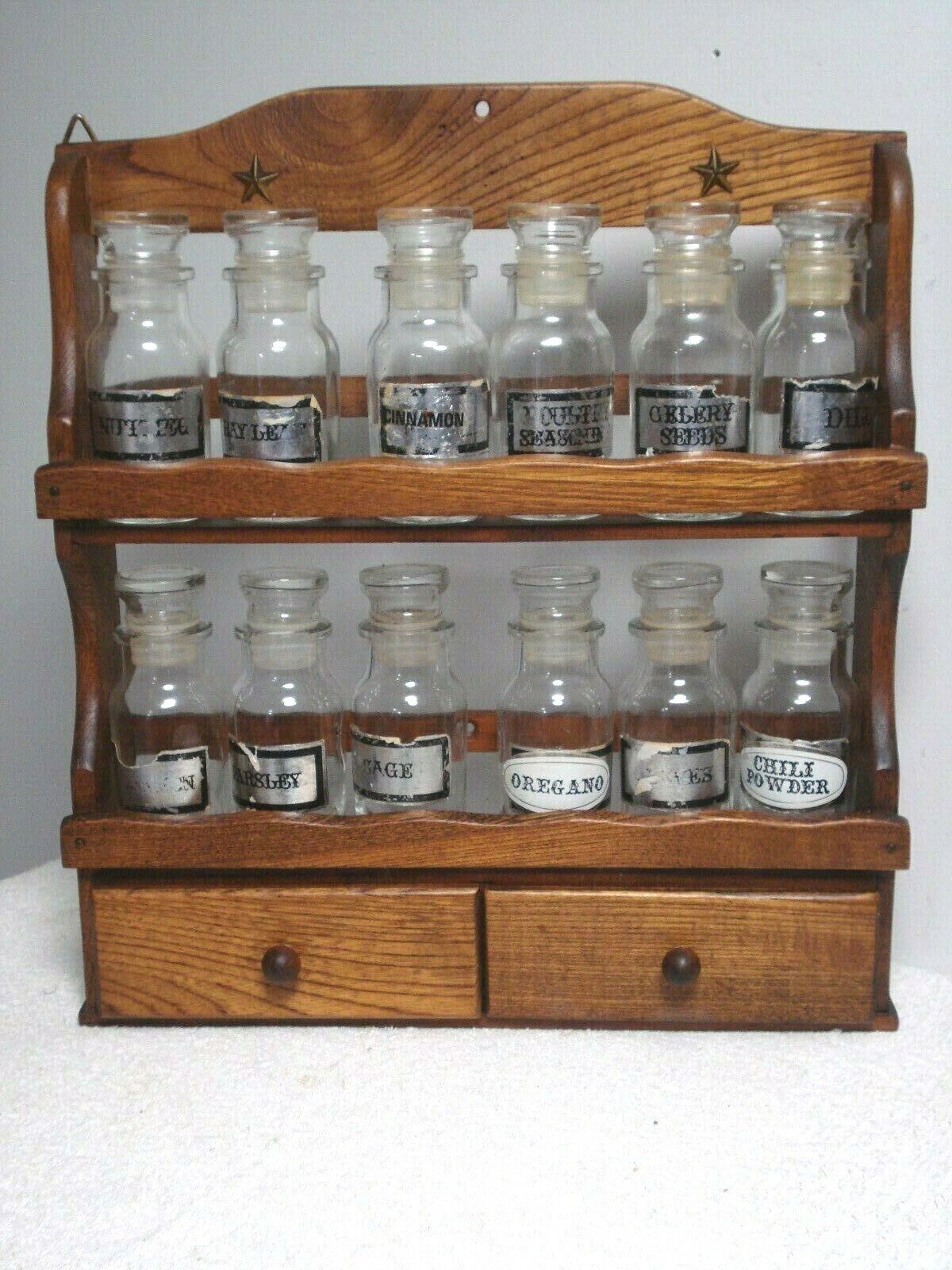This photograph showcases a wooden, wall-mounted spice rack with a rustic charm. The medium brown rack features two tiers, accommodating a total of twelve empty spice jars—six on the top shelf and six on the bottom shelf. Each jar bears a label, though some are more legible than others due to wear and age. Notable spices like cinnamon, celery seeds, chili powder, oregano, sage, and parsley are labeled, with some labels silver and others white. The structure includes two small drawers with wooden pull knobs positioned at the bottom left and right, slightly open and adding to the vintage appeal. The spice rack, suitable for kitchen use, also includes a couple of decorative stars at the top bracket and a central hanging hole, indicating it is designed to be mounted on a wall. The scene is set against a white surface and a blue background, enhancing the wooden texture of the rack, which might be made of refinished or stained oak.